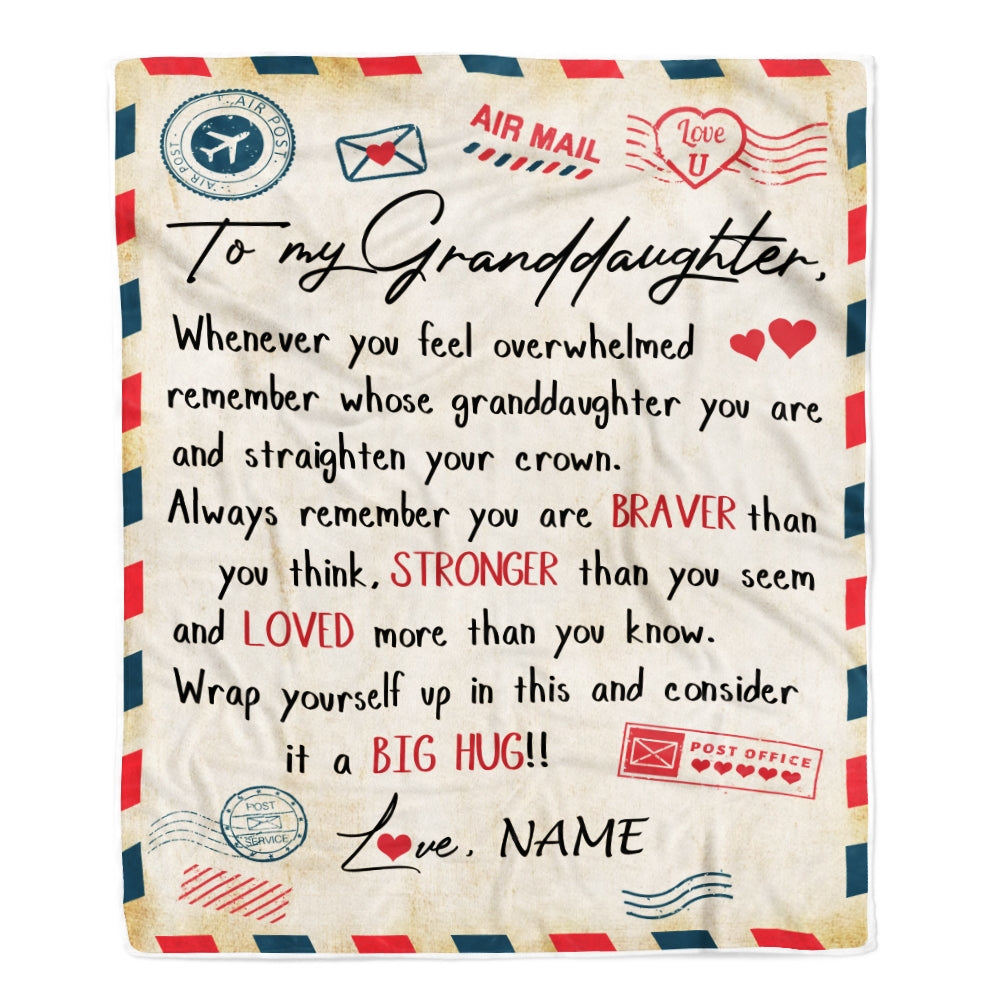The image showcases an aged letter with a brownish tint, indicative of its age. The edges of the photo are bordered with red, white, and blue colors, consistent with traditional airmail envelopes. In the upper left-hand corner, there is an air post stamp, suggesting it was sent via airmail. The letter is addressed to a granddaughter and contains the following heartfelt message in predominantly black ink: "To my granddaughter, whenever you feel overwhelmed, remember whose granddaughter you are, and straighten your crown. Always remember you are braver than you think, stronger than you seem, and loved more than you know. Wrap yourself up in this; consider it a big hug. Love, [Name]." Notably, the words "braver," "stronger," "love," and "big hug" are highlighted in red ink for emphasis. Additionally, there is a red ink postal stamp marking the letter.